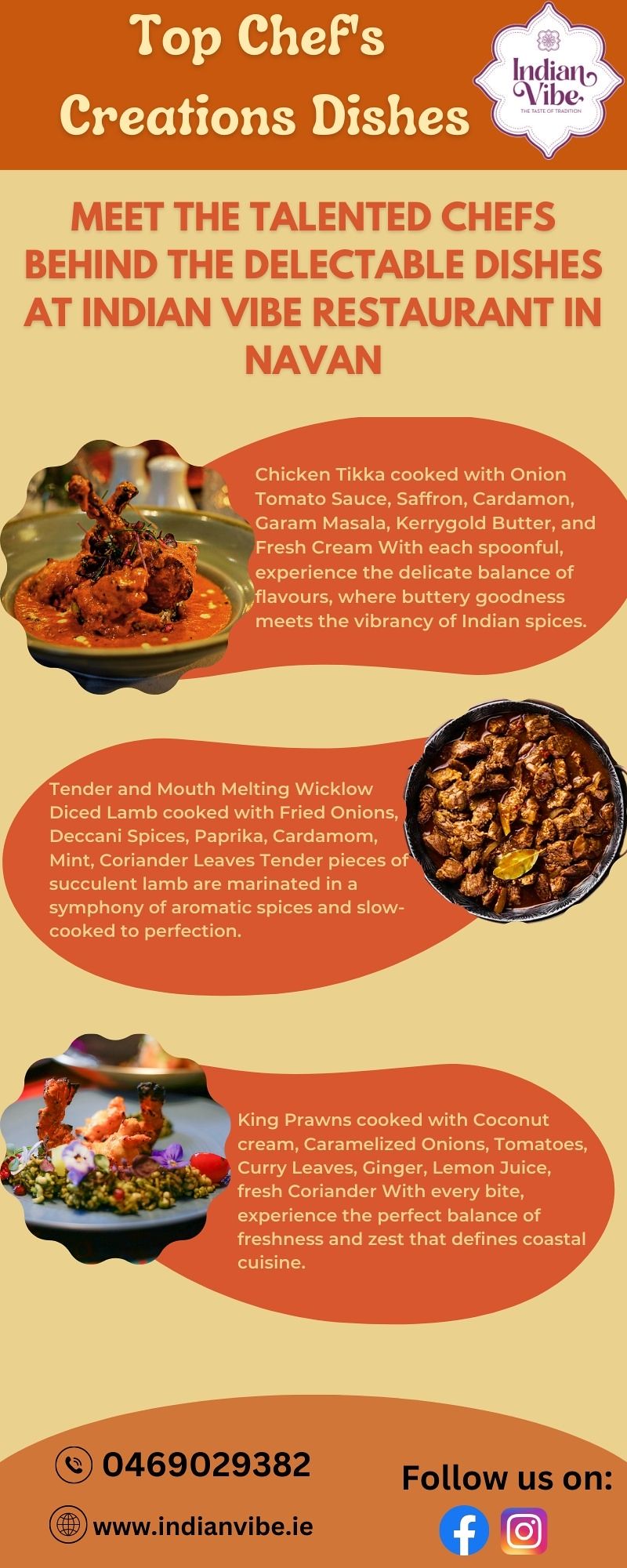This is a vibrant and appetizing advertisement for the Indian Vibe Restaurant in Navan, featuring "Top Chefs Creation Dishes." The ad, set against a yellow and orange background, introduces you to the talented chefs and their delectable creations. Highlighted with colorful images and detailed descriptions, it presents three standout dishes. The first is Chicken Tikka, cooked with onion, tomato sauce, saffron, cardamom, garam masala, Kerrygold butter, and fresh cream, creating a perfect balance of buttery richness and vibrant Indian spices. The second dish showcases tender, mouth-melting Wicklow diced lamb, prepared with fried onions, spices, paprika, cardamom, mint, and coriander leaves, slow-cooked to perfection. The third picture features king prawns cooked with coconut cream, caramelized onions, tomatoes, curry leaves, ginger, lemon juice, and fresh coriander. The ad, with its cheerful and engaging design, also includes contact information, a website, and social media links for further connection.